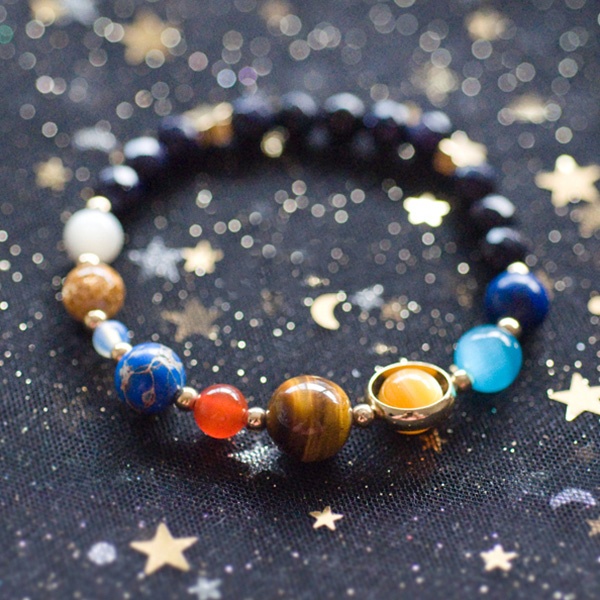This image is a close-up photograph of a bracelet, meticulously laid on a dark navy blue fabric adorned with gold glitter, small gold stars, and moons. The bracelet itself features a row of beads that are designed to represent the planets and celestial bodies. Among these beads, there's a yellow one symbolizing the Sun, a white bead, a blue bead representing Earth, and a small clear bead beside it for the Moon. There are also beads made from materials like tiger eye, carnelian, and lapis lazuli, interspersed with small round gold beads. The bracelet appears to be both artistic and thematic, drawing inspiration from the solar system, with the design elements creating a space-like aesthetic. The photograph has a sharp focus on the foreground, making the intricate details of half the bracelet and the rich, cosmic texture of the background cloth stand out, while the rest subtly blurs into the background.